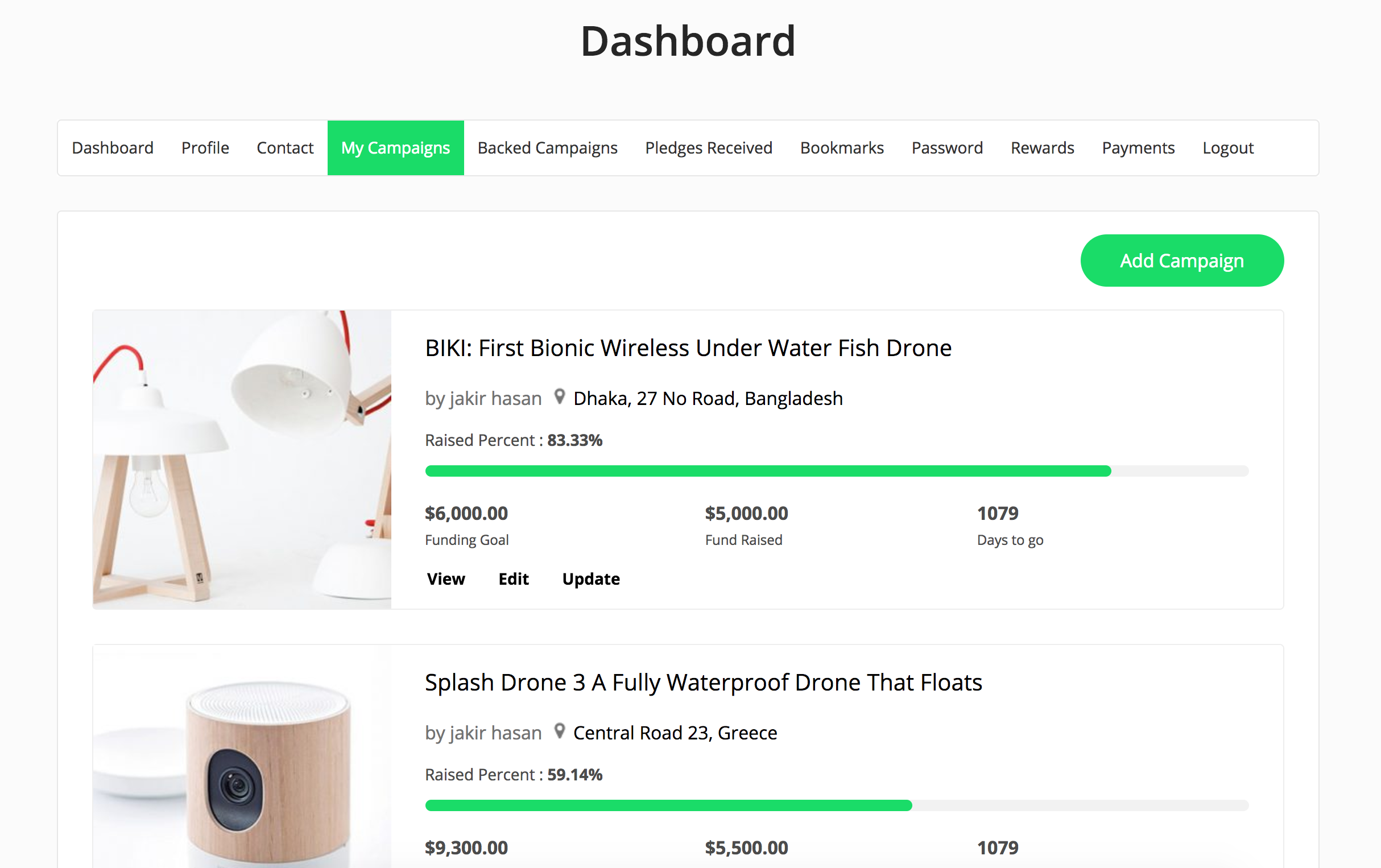The image displays a user dashboard on a white background. The dashboard profile includes options for "Contact" and "My Campaigns." In the highlighted green sidebar, the options listed are "Back Campaigns," "Pledges," "Received," "Bookmarks," "Password," "Rewards," "Payments," and "Logout." 

At the top right corner, there's a green circle with "Ad Campaign" written in white text. Below this, the user Bickey is managing two campaigns. 

The first campaign, titled "First Bionic Wireless Underwater Fish Drone," has successfully raised 83.33% of its $6,000 funding goal, amounting to $5,000, with 1079 days remaining. 

The second campaign is for the "Splash Drone 3, A Fully Waterproof Drone That Floats." This campaign has raised 59.14% of its $9,300 funding goal, totaling $5,500, also with 1079 days remaining. 

Both campaigns have options to "View," "Edit," and "Update."